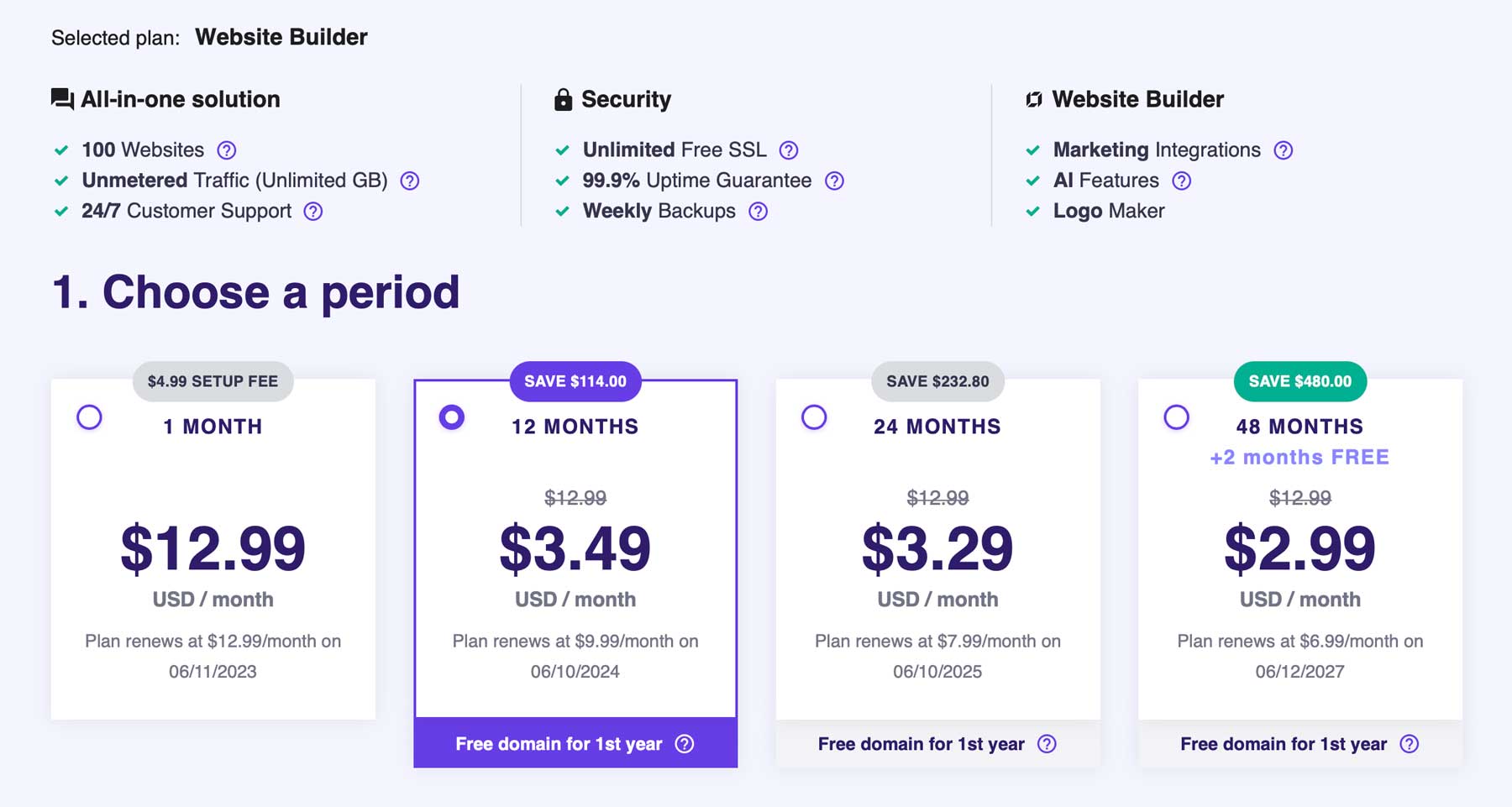This screenshot from a web page features a hosting plan selection interface set against a background of very light green. In the top left-hand corner, the selected plan is identified as "Website Builder." Below that, a list of plan features is displayed, including:

- All-in-one solution
- Support for 100 websites
- Unmetered traffic
- 24/7 customer support
- Unlimited free SSL
- 99.9% uptime guarantee

Further down, a prominent black font heading reads "Choose a period," accompanied by four pricing options in separate boxes. The options vary by duration:
- The one-month plan, priced at $12.99 per month, is the most expensive.
- The 48-month plan, priced at $2.99 per month, is the most cost-effective option.